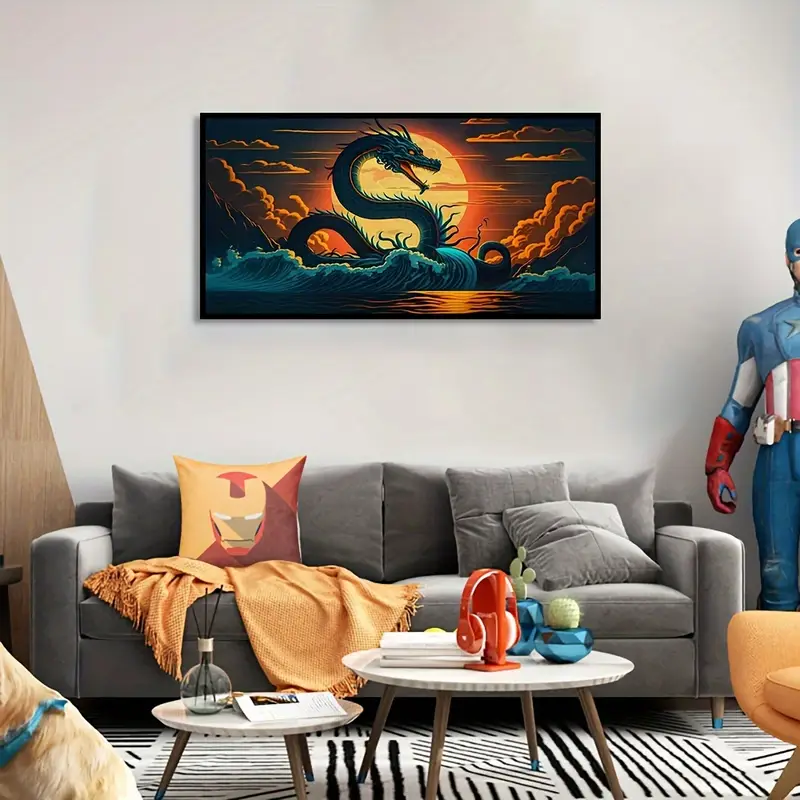This image depicts a living room with a vibrant, detailed mural as the focal point. The mural, approximately six feet long and three to four feet tall, features an S-shaped green dragon in front of a burning sun and an orange-tinted sky, with blue ocean waves and surrounding clouds, all framed elegantly in black. Below the mural, a gray felt-like couch is situated, adorned with three cushions: two that match the couch's gray color and a third featuring Iron Man's face set against a red and yellow background. A golden throw blanket is draped over the couch near the superhero-themed cushion.

In front of the couch are two white, circular coffee tables of different heights. The taller table holds a pair of red headphones, two blue vases with cacti, and a stack of paper. The shorter table supports an open book and a decorative bottle-shaped globe holding three black sticks. Below the tables, a black and white striped rug, featuring a mix of vertical and zigzag lines, spreads out across the floor.

In the bottom left corner of the image, partially captured, is a Labrador retriever with a blue bandana around its neck. To the right of the couch, a life-size Captain America action figure stands prominently, though only part of it is visible. Additionally, the bottom right corner of the image reveals an orange armchair, only partially in the frame.